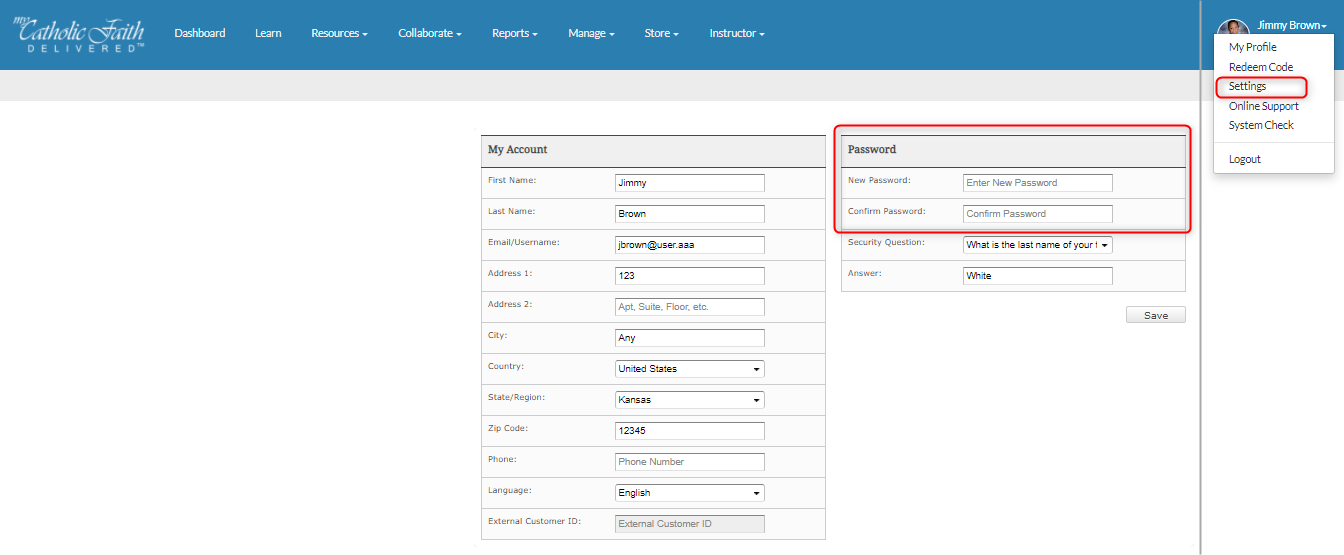The image portrays a detailed screen interface of the "Catholic Faith Delivered" platform. At the top, there is a blue navigation bar on the left side with menu items in white text, including Dashboard, Learn, Resources, Collaborate (with a drop-down), Reports (with a drop-down), Manage (with a drop-down), Store (with a drop-down), and Instructor.

The account information section for the user "jimmybrown" (jbrownuser at AAA) is displayed prominently. Due to placeholder text, details such as Address 1 (123), Address 2 (suite floor, etc.) remain unspecified. The City is listed as "Any," with the Country drop-down set to USA and the State/Region set to Kansas. The Zip Code field contains "12345," and the Phone Number field is grayed out. The Language drop-down is set to English, while the External Customer ID field is empty.

To the right, a section designated for updating the password is highlighted with a red rectangle, covering the fields for Password, New Password, and Confirmed Password. Below this section, a security question is posed, asking for the last name with a drop-down for specific queries and an answer field set in white.

At the bottom of the interface, there is a "Save" button. A pop-up menu is visible, containing options such as My Profile, Redeem Code, Settings, Online Support, System Check, and Log Out. The Settings option is marked with a red triangle, suggesting it is of particular importance, potentially for educational use.